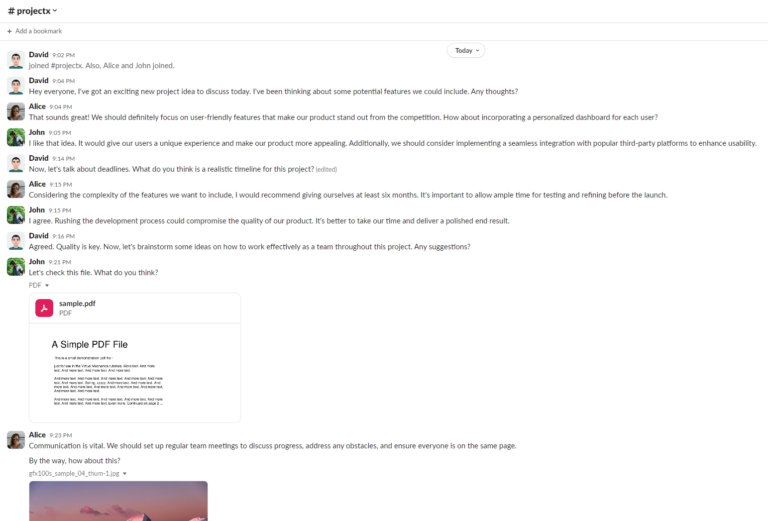The screenshot captures a dynamic conversation on a collaboration platform, focused on the development of a computer application known as "Project X." Displayed on a clean white background with black text, the conversation unfolds in a vertical column involving three individuals: John, David, and Alice. 

At the top left, the text "Project X" is prominently featured in black, accompanied by a pound symbol. A downward-facing arrow appears next to the project name, suggesting additional options for managing the project. Below that, in gray text, the phrase "add a bookmark" is shown alongside a plus symbol, indicating the ability to bookmark the conversation.

The dialogue spans from 9:02 p.m. to 9:23 p.m., documenting a 21-minute exchange. Throughout the conversation, the participants discuss various aspects of the project, including desirable features, development strategies, and scheduling future meetings. 

The timestamps accompanying each message mark the flow and pace of the discussion. Alice concludes the conversation at 9:23 p.m. with a statement emphasizing the importance of regular communication: "Communication is vital. We should set up regular team meetings to discuss progress, address any obstacles, and ensure everyone is on the same page." Additionally, she attaches an image, likely a concept art or design proposal relevant to the project.

Overall, the screenshot illustrates a collaborative effort where ideas are shared, tasks are coordinated, and clear communication is maintained to propel the project forward.